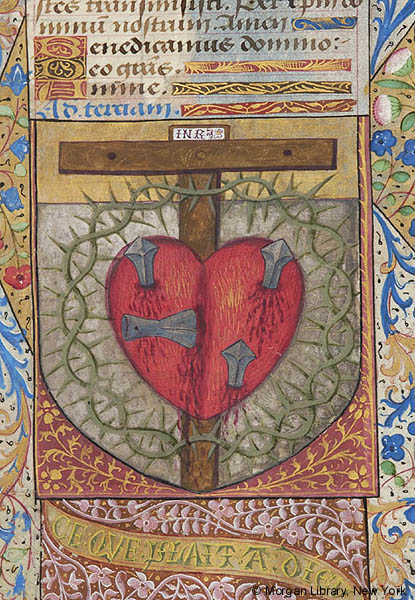This detailed artwork emulates a medieval renaissance style and prominently features a striking central image of a heart impaled by four silver metal spikes, mounted on a T-shaped, brown wooden cross. Encircling the heart is a crown of thorns, adding to its intense visual impact. The central imagery is framed by an intricate gold floral design shaped like a 'U' and set against a rich red background. Below this central motif, a pink flowery pattern adorns the red backdrop, leading to a banner inscribed with unreadable text. The sides of the image are bordered by colorful floral designs in hues of blue, green, gold, and red, enhancing the ornate appearance. At the top, there are five layers of text, likely in Latin, further contributing to the historical feel. The piece is marked with a copyright in the bottom right corner, stating "Morgan Library, New York." This detailed composition resembles a poster with its layered textual and visual elements, symbolizing themes of love and sacrifice.